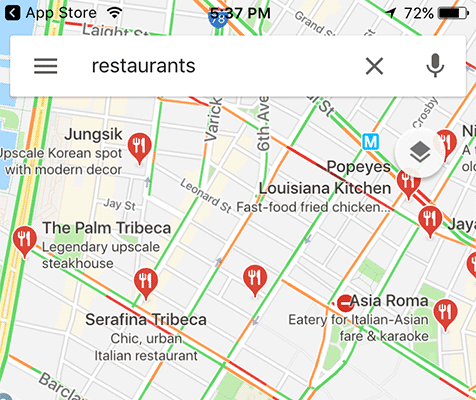This image features a detailed map showcasing various locations primarily in the Tribeca neighborhood. Highlighted spots include notable establishments such as Junksik, Lipalm, and multiple mentions of Serafina and Tribeca. Other prominent points of interest are Chick, Urban Italian Restaurants, Asia Roma, E3 – a venue for Italian, Asian cuisine and fairs, and Karaoke. Additionally, Louisiana Kitchen is marked, known for its fast-food fried chicken. Puppies, Leonard Street, 6th Avenue, Crosby Street, and Grand Street are also identified. The map is visually colorful, utilizing shades of blue, black, and red to distinguish these locales. Several map pins, illustrated with a fork and knife, indicate restaurant locations. The image also features a search field incorporating these colors for aesthetic coherence.